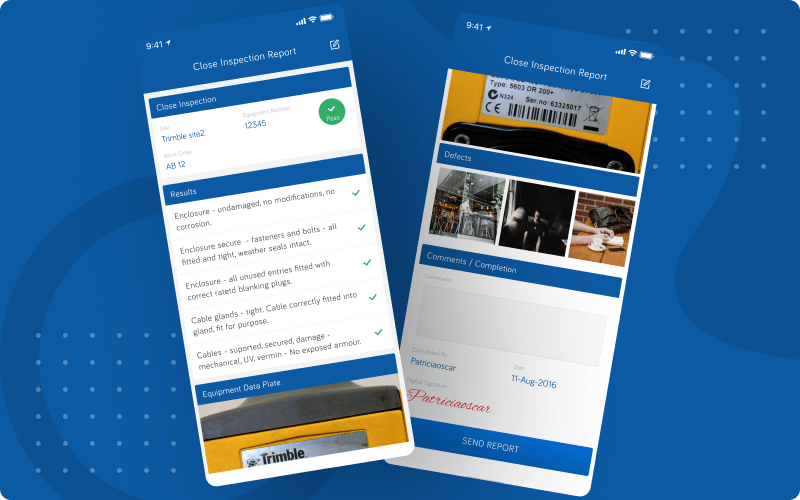This rectangular image, which is about 50% wider than it is tall, features rounded edges that add a unique touch to its design. The background exhibits a gradient transitioning from medium blue to dark blue, creating various shapes and angles that play with the viewer's perception. Notably, a dark blue circle rests in the lower-left corner while a swirling wave-like pattern separates the different shades in the upper-right corner.

Overlaying this visually intriguing backdrop are two clear cell phone screenshots. At the top of each screenshot, typical status bar indicators—such as time, signal strength, and battery level—confirm their origin as mobile devices. The top 20% of the screenshots sport a medium blue background with white lettering that reads "Close Inspection Report," accompanied by an edit button on the right.

Beneath this title on each screenshot is a similarly-colored bar labeled "Close Inspection." Although the specific text within these bars is unreadable, they are divided into three distinct sections, suggesting a detailed inspection report segmented for clarity.